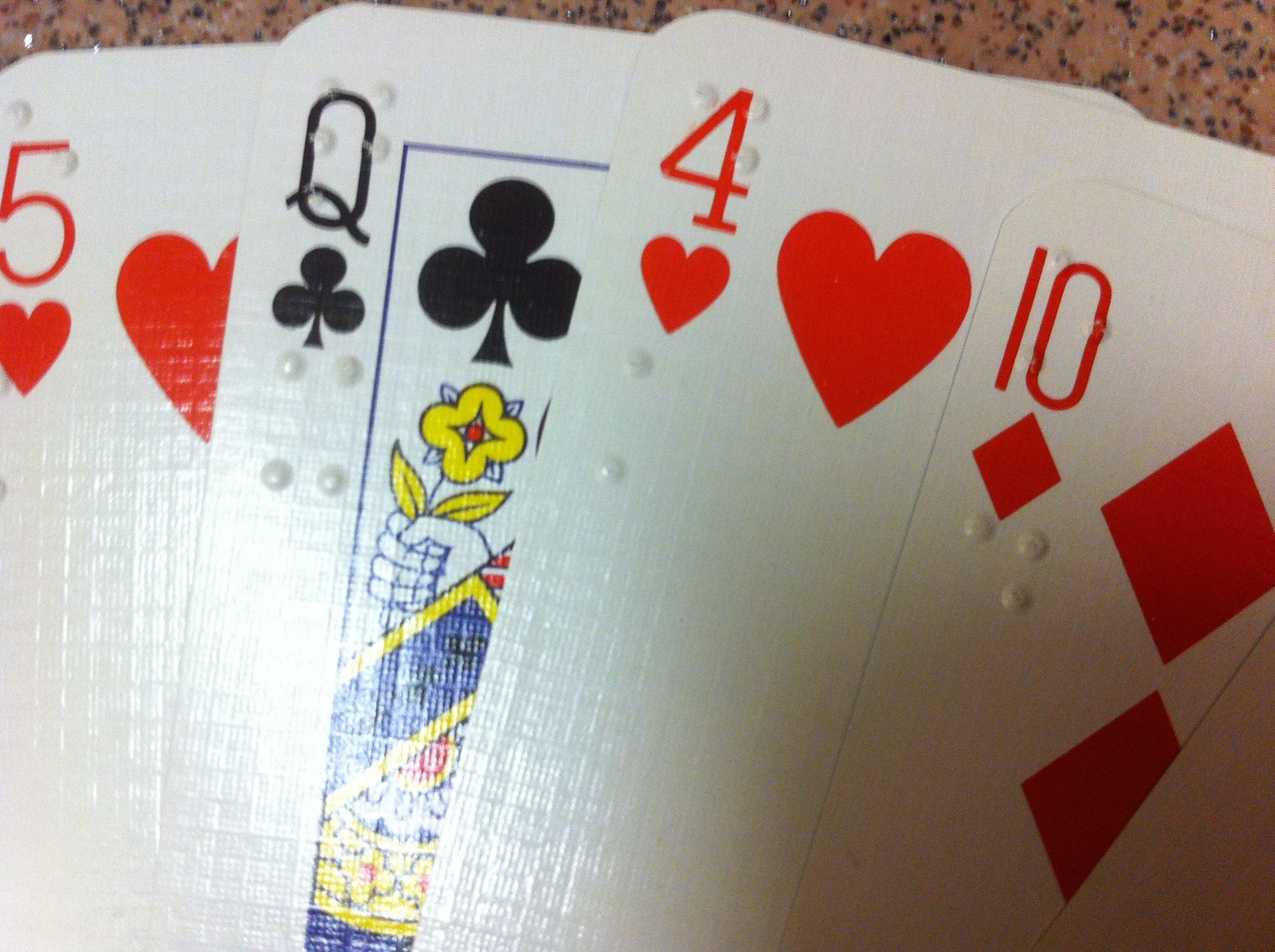This color photograph is a close-up of four playing cards meticulously arranged on a brown and black granite or Formica-style surface. From left to right, the cards displayed are: the five of hearts, the queen of clubs, the four of hearts, and the ten of diamonds. The five of hearts card features a red numeral ‘5’ at the top left corner, a red heart symbol below, and a partial red heart along the side. The queen of clubs card showcases a black letter ‘Q’ and a club symbol, along with a fragment of the card's central artwork, which includes a black club, a hand holding a yellow and red flower, and part of the queen's robe, although the queen herself is not visible. The four of hearts card displays a red numeral ‘4’ and a heart symbol below it, along with a larger red heart to the right. The ten of diamonds card features a red numeral ‘10’ and a diamond symbol underneath it, with two partial red diamonds visible to the right. A fifth card is partially visible at the bottom right corner, but its identifying marks are not discernible. Notably, each card is embossed with raised dots, suggesting they are marked with braille for accessibility.